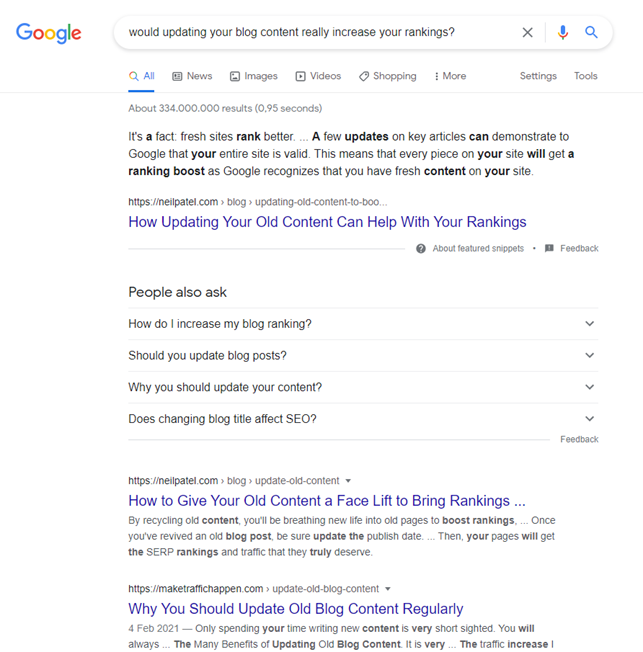This is a detailed description of a screenshot of a Google search results page. At the top, the Google search bar displays the query: "Would updating your blog content really increase your rankings?" Directly below the search bar, the results summary states: "About 334,000,000 results (0.95 seconds)." 

Above these results, the Google toolbar is present, featuring standard tabs: "All," "News," "Images," "Videos," "Shopping," as well as the additional options "More," "Settings," and "Tools."

The first search result is prominently displayed and emphasizes the importance of fresh content. It reads: "It's a fact. Fresh sites rank better. A few updates on key articles can demonstrate to Google that your entire site is valid. This means that every piece on your site will get a ranking boost as Google recognizes that you have fresh content on your site."

Below this, additional search results are listed, each with blue hyperlinks indicative of clickable links. The second result is titled: "How updating your old content can help with your rankings." The third result reads: "How to give your old content a facelift to bring rankings." This is followed by a fourth result: "Why you should update old blog content regularly," which includes a brief description beneath the title.

Each search result is separated by subtle lines, helping to delineate the individual entries. The results offer a range of advice and insights into the benefits of updating blog content to improve search engine rankings.